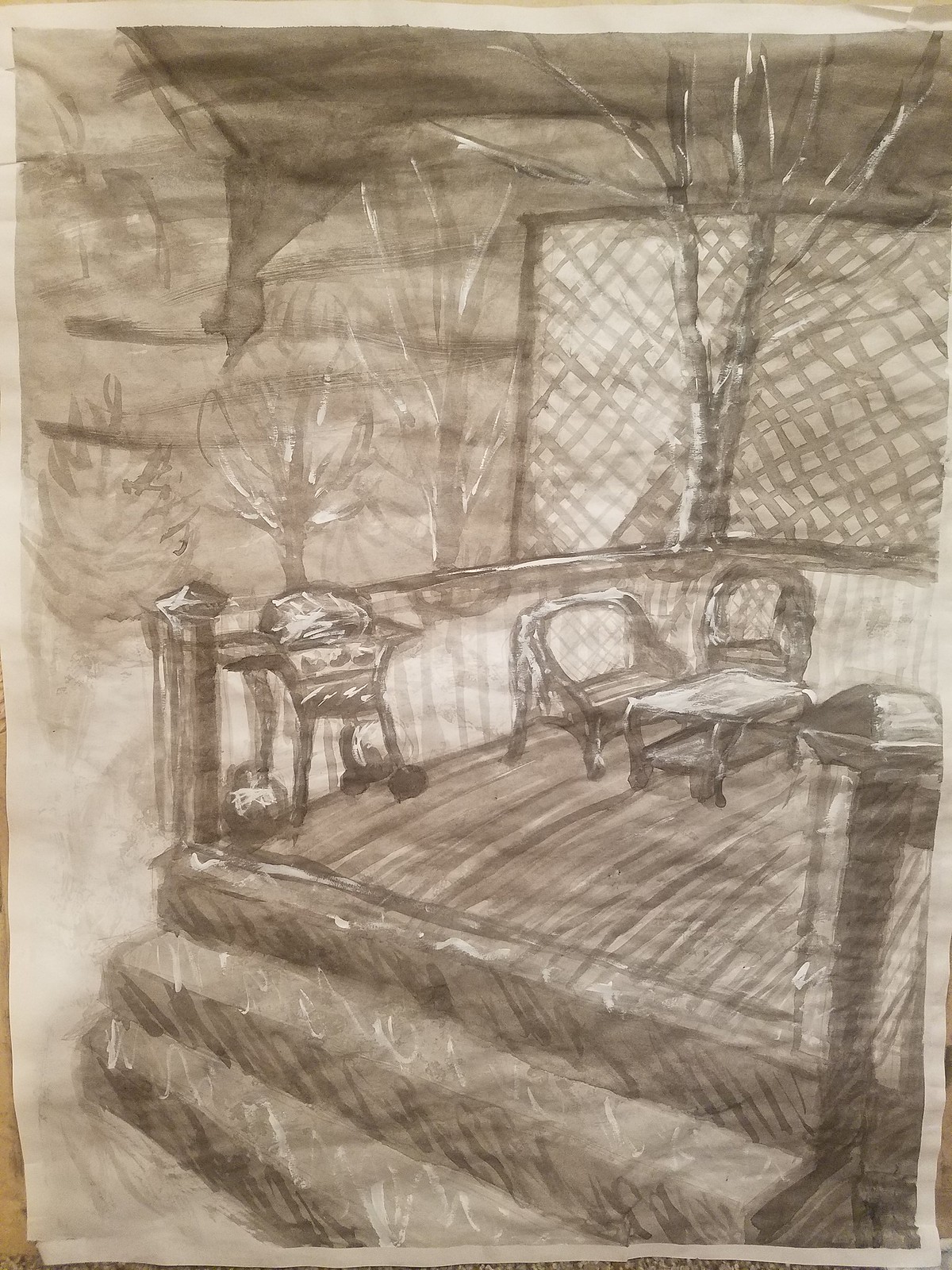The rectangular, vertically-aligned image showcases a meticulously detailed pencil sketch on sepia-toned paper, capturing the serene and rustic essence of a wooden porch. The illustration depicts a three-step porch characterized by its traditional wooden slat construction. On the porch, arranged from left to right, a barbecue grill leans casually against the railing, evoking the promise of cozy outdoor gatherings. Centrally positioned, a chair with a low table in front of it offers a quaint seating area, inviting contemplation or conversation. 

Beyond the porch railing, a lattice fence rises, partially obscured by the slender trunk of a small, leafless tree, which adds a touch of stark beauty to the composition. The scene above contrasts dramatically with the calm setting below: a menacing, swirling tornado descends from dark, ominous clouds, its narrow funnel pointing precariously towards the serene porch. This juxtaposition of tranquility and turmoil brings an evocative depth to the artwork, making it a strikingly atmospheric piece.